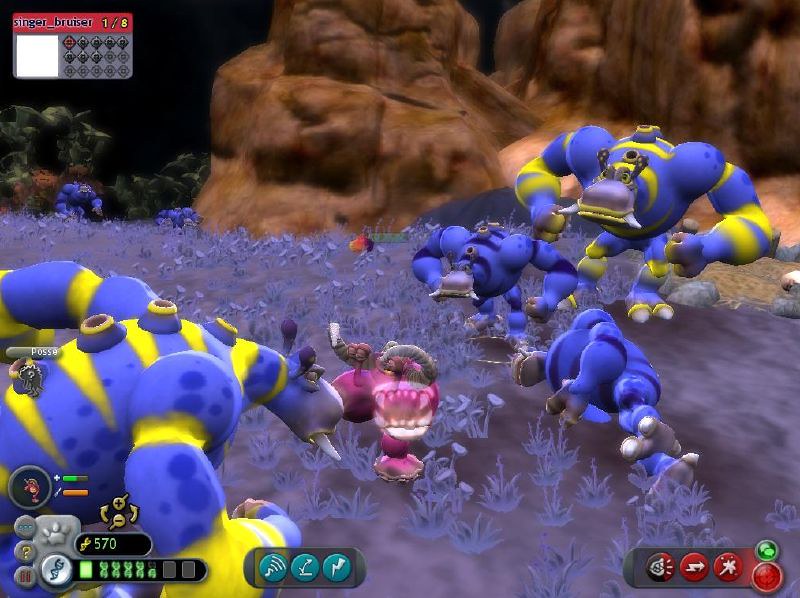The image is a slightly wider-than-tall screenshot from an early 2000s or late 90s video game, presented in a third-person, open-world style. The bottom two-thirds of the scene features a purple terrain dotted with long, narrow, fern-like leaves, suggesting an alien or fantastical environment. In the foreground, a cluster of humanoid creatures are depicted, including four blue monsters and a singular pink monster at the center of the conflict. The blue monsters, some larger with yellow stripes and others smaller with darker blue stripes, also exhibit distinct features like protrusions and colored rings along their spines. The pink monster, significantly smaller, has big teeth and horns, presenting as the protagonist caught in the midst of a chaotic battle. The terrain is bordered by out-of-focus brown boulders and cliffs, contributing to the otherworldly atmosphere. The user interface includes a health and inventory display at the bottom, as well as a heads-up display on the top left, marked by text like "singer_bruiser," which further hints at the unique elements of the gameplay.